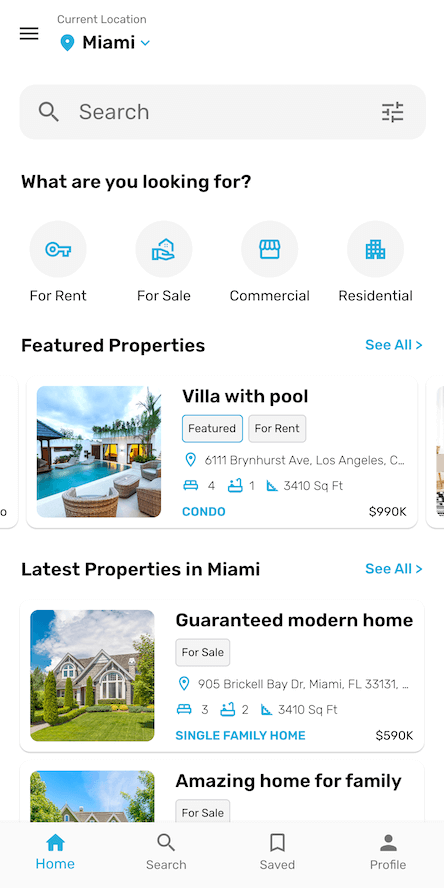A comprehensive screenshot of a real estate search interface set against a teal background. At the top, the location is identified as Miami, with a blank search bar underneath prompting, "What are you looking for?" To the right of the search bar, options for property types include a key icon labeled "For Rent," a hand holding a house icon labeled "For Sale," a building silhouette for "Commercial," and tall buildings for "Residential."

Further down, a section titled "Featured Properties" showcases detailed listings. The first is a luxurious villa with a pool, described as a condo located in Los Angeles, California, listed for $990,000. Below that is another featured property in Miami, labeled as a "Guaranteed Modern Home," promoted as an "Amazing Home for Family."